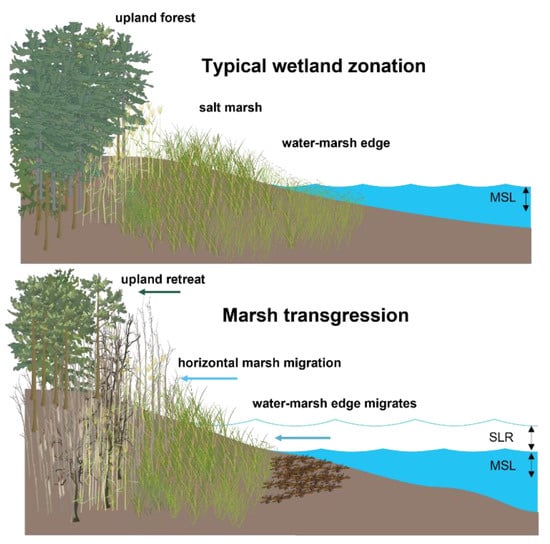The image features two horizontally aligned diagrams, one above the other, illustrating wetland zonation and migration. The top diagram is labeled "Typical Wetland Zonation" and shows a landscape with various vegetations. Near the top, it shows an "Upland Forest" transitioning into a "Salt Marsh," and finally a "Water Marsh Edge" adjacent to the blue water labeled "MSL" (Mean Sea Level). The vegetation includes trees, grasses, and other foliage on a sandy terrain leading down to the water.

The bottom diagram, labeled "Marsh Transgression," depicts similar terrain but with changes to the vegetation and landscape. It includes labels such as "Upland Retreat," "Marsh Transgression," and "Horizontal Marsh Migration." There are arrows pointing left, indicating the shift of these marsh areas. The "Water Marsh Edge" is also labeled as migrating and is affected by "SLR" (Sea Level Rise), shown through a wavy outline on the water's edge. This diagram suggests a dynamic environment with vegetative shifts and loss, with dead trees and changing water levels.